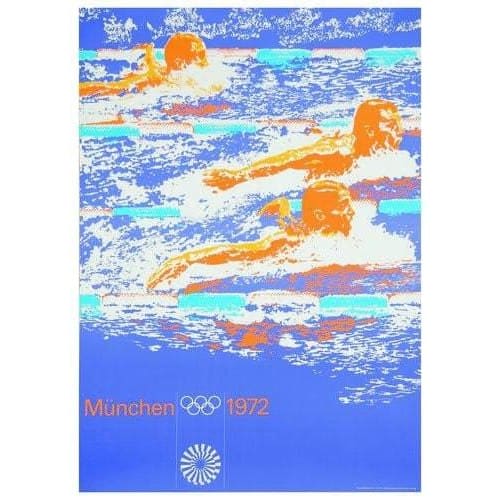This image is an abstract, vintage Olympic poster from the 1972 Munich Olympics. Dominated by muted hues, it prominently features the iconic interlocking five Olympic rings and the word "München," detailed with German umlauts. At the center of the composition, three orange-colored swimmers are depicted mid-competition, gliding towards the right within distinct lanes separated by turquoise barriers in periwinkle-colored water. The backdrop blends elements reminiscent of both sky and water, contributing to an overall artistic and somewhat surreal ambiance. At the bottom, the poster features two significant symbols: the recognizable five-ring Olympic logo, and a unique spiral shape. This visual is a captivating blend of sport and art, capturing the dynamic energy of the historic 1972 Olympic Games.